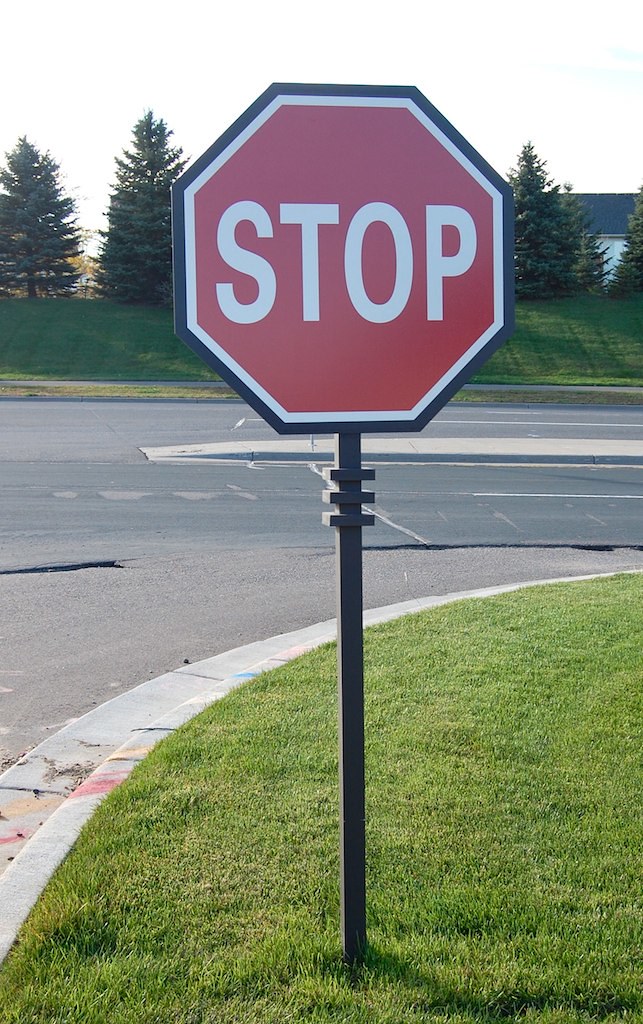This color photograph captures a neighborhood street corner on a clear day with a light grey sky and a few puffy clouds. The foreground is dominated by a prominent stop sign, mounted on a thick black metal pole, standing on neatly trimmed, short green grass. The stop sign is the typical red hexagon with large white letters that spell "STOP," outlined with a black metal frame. Surrounding the area is a silver grey curb. The scene extends to a two-lane road in each direction, separated by a concrete divider strip in the middle, suggesting it might be a four-lane street. In the background, gently rolling green grass covers a small hill adorned with rows of tall evergreen trees. Additionally, hinting at a residential area, rooftop hints and sizable trees are visible, completing this serene suburban landscape.